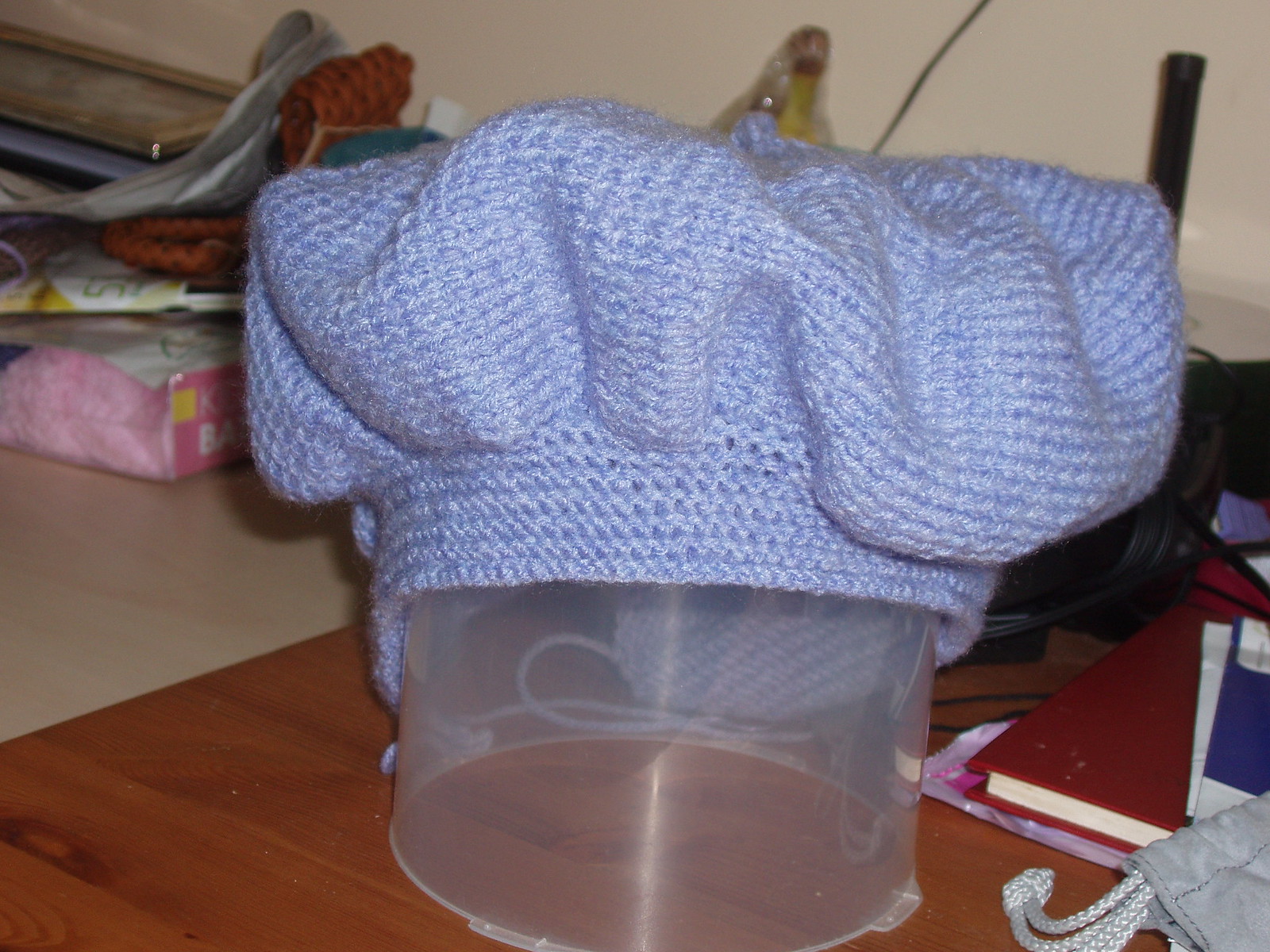This photograph showcases a light purple, knitted or crocheted hat modeled after the shape of a chef's hat, with a puffy top and a tight rectangular band at the bottom. The hat's intricate, fine-grained knitting pattern suggests a high level of craftsmanship, with each stitch appearing tight and well-executed. Perched on top of a clear plastic container, which sits atop a faux brown wooden desk, the hat is clearly visible. The setting is cluttered, featuring various indistinguishable objects and projects, along with a hard-to-distinguish red-covered hardcover book on the right. The background displays a tan or creamy white wall. Other notable items include a pack of tissues, headphones, and books, adding to the overall impression of a busy, cluttered workspace.